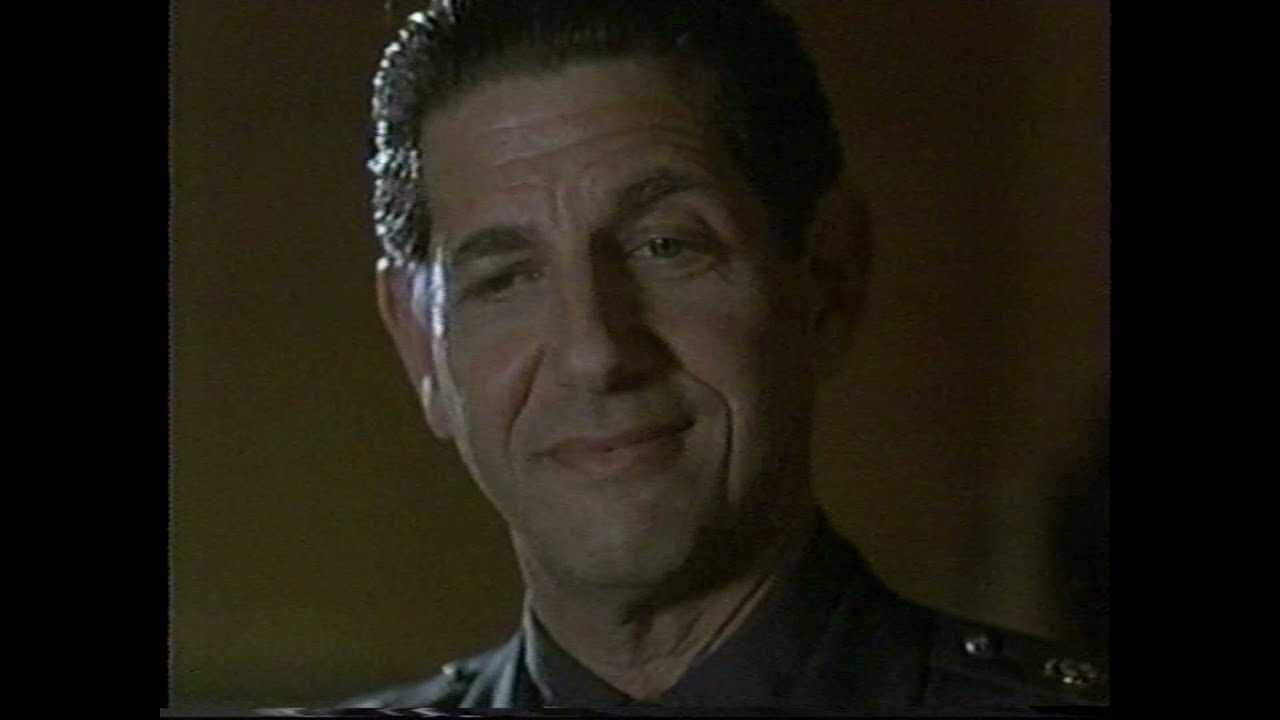The image is a still shot from an older movie or TV show, presented in color but noticeably grainy. It features a close-up of a middle-aged Caucasian man with a light complexion and short, slicked-back dark brown or black hair. His expression is focused and intense, with a tight-lipped smile and lines across his forehead. His eyes are open and directed downwards towards the lower left of the screen, and his left eyebrow is slightly raised. The man is wearing a dark gray or black uniform adorned with metallic pips on the shoulders, though the exact details are partially obscured since the image only captures him from the top of his shoulders to his slightly cropped head. The background is blurred and predominantly brown, possibly depicting a wall, lending an indistinct and nondescript setting. Thick black borders frame the image on the left and right sides, emphasizing its cinematic origin. The overall ambiance suggests a poised moment of contemplation or anticipation.